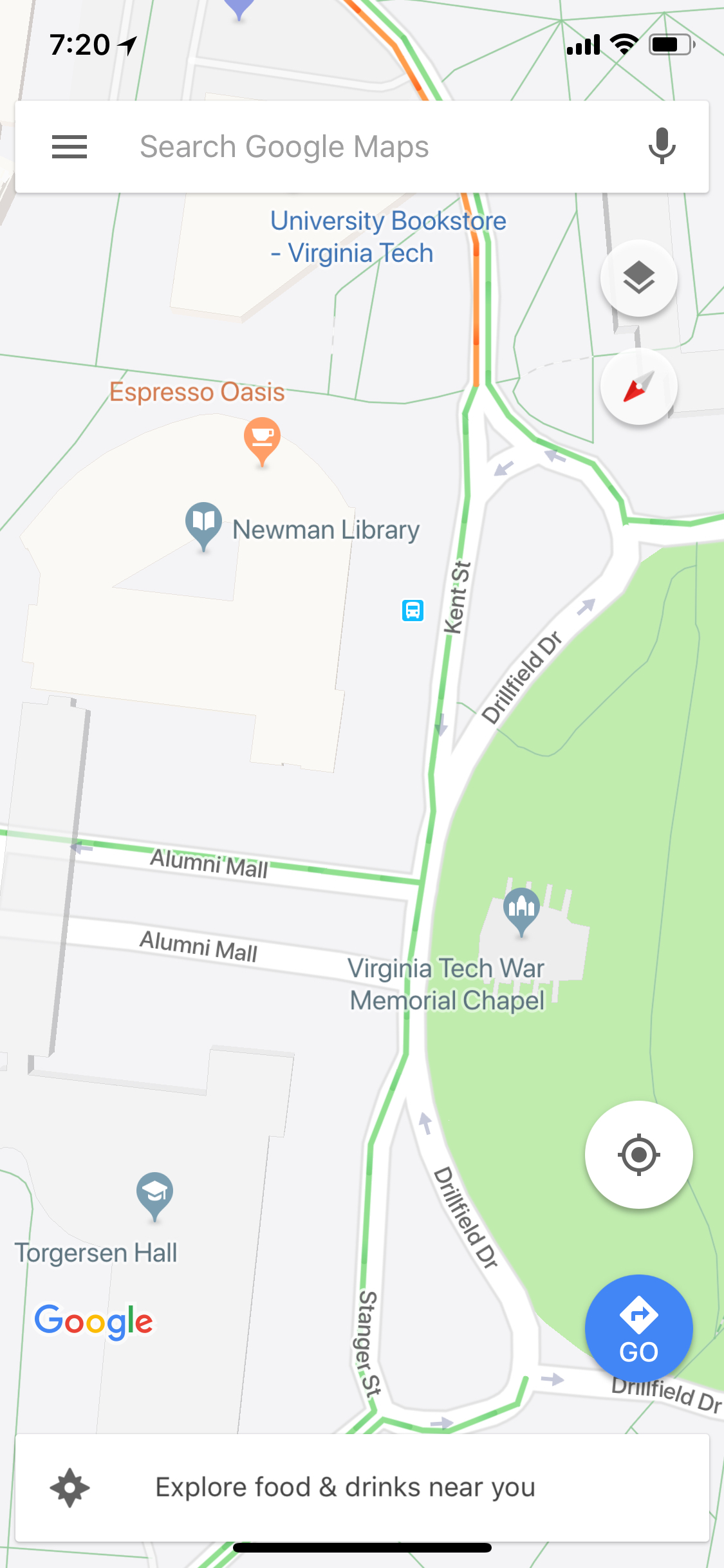The image depicts a screenshot of the Google Maps app interface. At the top, it displays a status bar showing "720" with an airplane-mode icon, four black graduated bars indicating signal strength, a Wi-Fi symbol, and a battery icon filled to three-quarters capacity. Below the status bar, there is a white search box containing three horizontal stack lines for the menu, the text "Search Google Maps" in gray, and a microphone icon to the right for voice search.

The map view itself features prominent landmarks and streets including the "University Bookstore," "Virginia Tech" highlighted in blue, and roads such as "Kent Street," "Drillfield Drive," and "Alumni Mall." Significant buildings like the "Virginia Tech War Memorial Chapel," "Torgersen Hall," "Newman Library," and "Expresso Oasis" café are also labeled on the map.

At the bottom of the screen, a white banner with a compass icon prompts, "Explore food & drinks near you." In the bottom right corner, a cluster of interactive buttons appears; a white circle with the location symbol for centering the map, and a blue circle with a white diamond background and an arrow pointing to the right, labeled "Go," designed for initiating navigation.